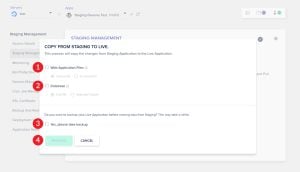This is a small, blurry image primarily composed of text that is difficult to read. The only discernible words are "copy from" and a partially legible segment that appears to either be "to live" or "to live." Within the image, there are red circles numbered sequentially from 1 to 4. Additionally, there is a white rectangle in the center featuring the word "Cancel" in black letters. The image contains no photographic or pictorial elements such as people, animals, plants, buildings, or vehicles.